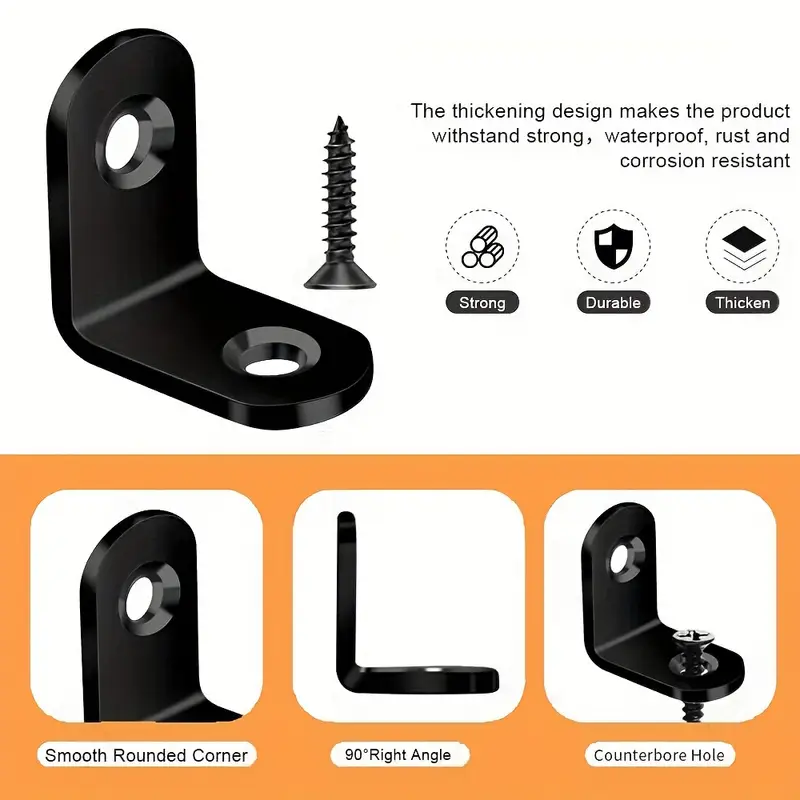This detailed instructional image serves as both a tutorial and advertisement for a sturdy L-shaped bracket. The top half features a prominent, enlarged computer-generated graphic of a dark black bracket accompanied by a screw. Adjacent text highlights the bracket's thickened design, boasting its ability to withstand strong forces, waterproof conditions, and resist rust and corrosion.

To the right of this main image, icons emphasize the bracket's key features: strength, durability, and thickened design. Below, three zoomed-in visuals are presented within orange frames: one shows the smooth, rounded corner of the bracket; another illustrates the 90-degree right angle; and the third displays the counterbore hole for screw insertion.

The diagram is clear and user-friendly, showcasing the bracket's practical applications, such as reinforcing furniture, cabinets, or drawers at a right-angle joint for increased stability and strength.